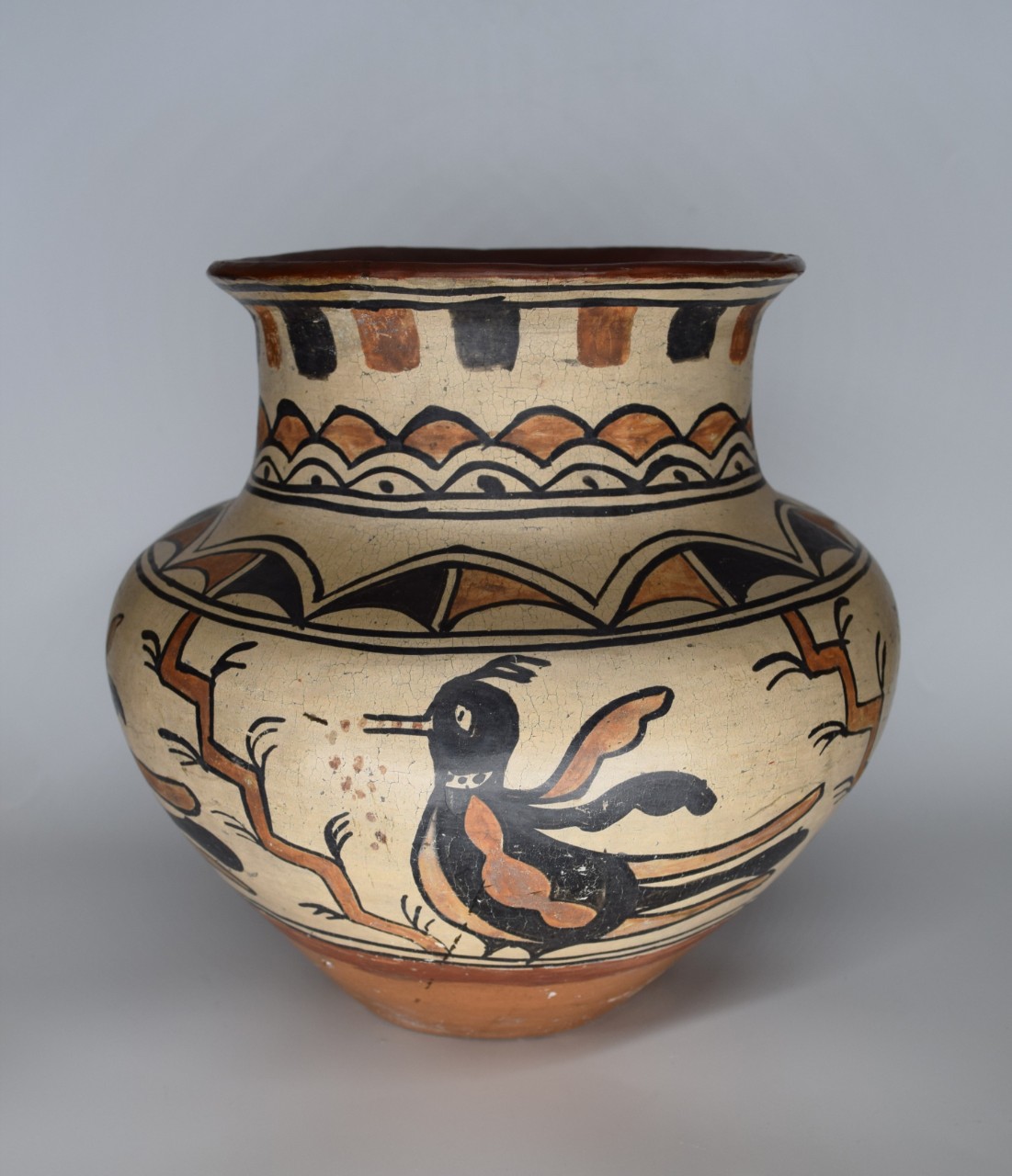The image features a vertically aligned ceramic vase, likely an old artifact, situated on a mid-gray surface that serves as a consistent backdrop. The vase itself showcases a sophisticated blend of colors and artistic details. The base starts with a medium brown color, seamlessly transitioning into a primarily tan background with darker shades of brown and burnt orange hues that provide a rich contrast.

The vase’s shape features a wide, rounded bottom that narrows towards the top, reminiscent of a traditional water jug. Prominent on the lower portion of the vase is an intricate illustration of a bird facing left, rendered in dark brown and black with lighter brown wings. The bird is characterized by a couple of dark brown feathers sprouting from its head. Surrounding the bird are textured, zigzag lines that morph into branch-like patterns with leaves, all in varying shades of brown and burnt orange.

As the vase starts to narrow, decorative semi-circular and oval patterns emerge, culminating at the top with a series of alternating dark brown and medium brown square accents around the rim. This detailed mix of artistic elements and earthy colors highlights the vase’s historic and cultural significance.